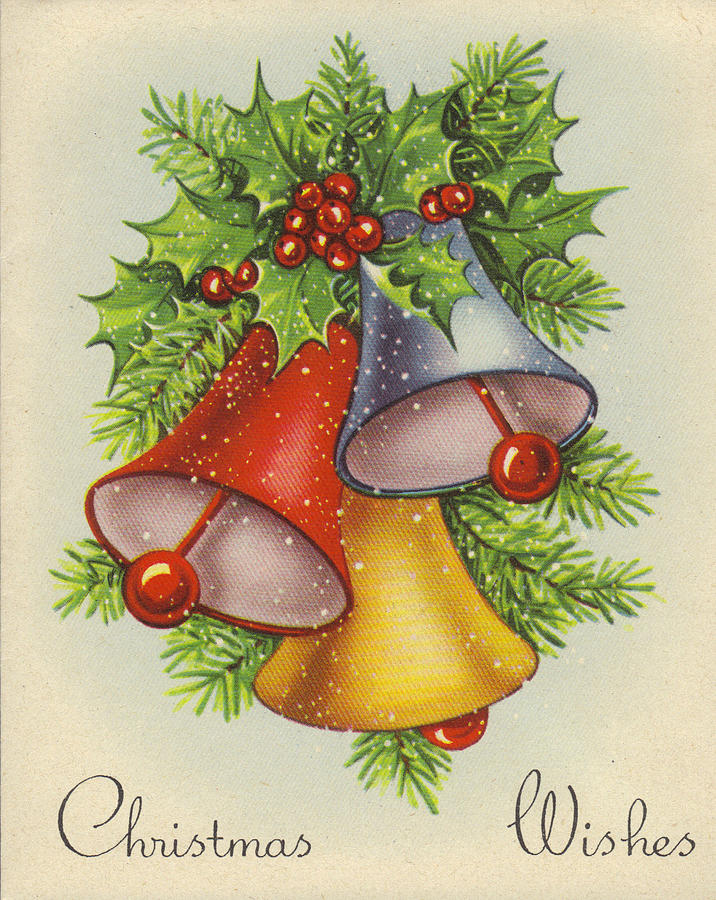The image appears to be the front of a festive, old-fashioned Christmas card featuring a detailed artistic illustration. Centered in the design are three jingle bells arranged vertically: a blue bell at the top, a red bell in the middle, and a yellow bell at the bottom. All the bells have red clappers. Surrounding the bells are lush green foliage, including holly with red berries and evergreen branches. The background is a muted light beige-blue color, adding to the vintage appearance of the card. Over the image, white splatter mimics softly falling snow. At the bottom, the cursive inscription "Christmas Wishes" is written in a greyish-black font, evoking a nostalgic feel.